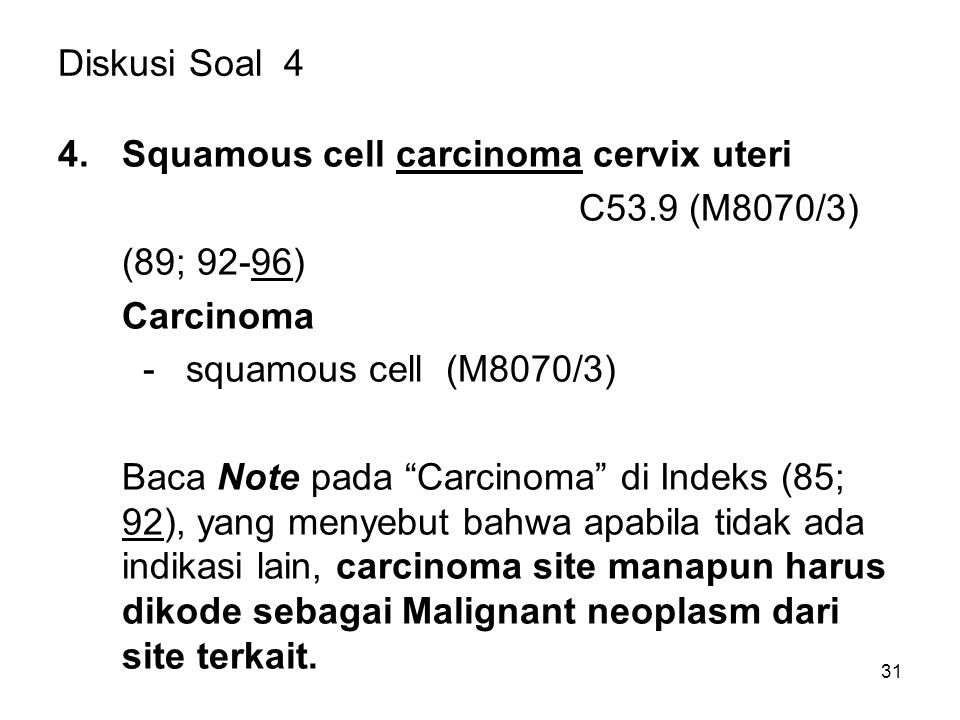The image depicts a page from a book or reference guide, featuring text predominantly in black and white. At the top, the heading reads "Disclusive Soul 4," followed by the numeral "4." Below this, it states "Squamous Cell Carcinoma Cervix Uteri," with the medical classification "C53.9 (M8070/3)" underneath. The subsequent lines include the numbers "89, 92-96," and the term "carcinoma" in bold font. Further down, it mentions "squamous cell (M8070/3)" followed by the abbreviated term "BACA," and then "note" in bold. The final section comprises a definition or description written in a different language, spanning a total of five lines. The layout suggests it could be an encyclopedic entry or part of a medical dictionary.